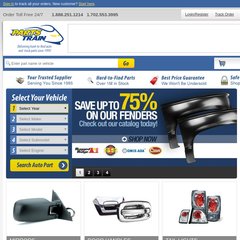A heavily blurred and pixelated screenshot displays a webpage from Pulse Train, a website primarily featuring a white and dark blue color scheme with accents highlighted in yellow text or text boxes. Despite the blurred elements, the website’s layout suggests a 24/7 operational model, possibly offering free delivery. Prominently advertised are guarantees of the best prices and partnerships with trusted suppliers. 

A key feature allows users to search for vehicle-specific parts by entering their number plate. The screenshot indicates active promotions, such as a 75% discount on fenders, prominently displayed in the central area. Towards the bottom, the website showcases images of various car parts, including door locks, door handles, wing mirrors, and brake lights.